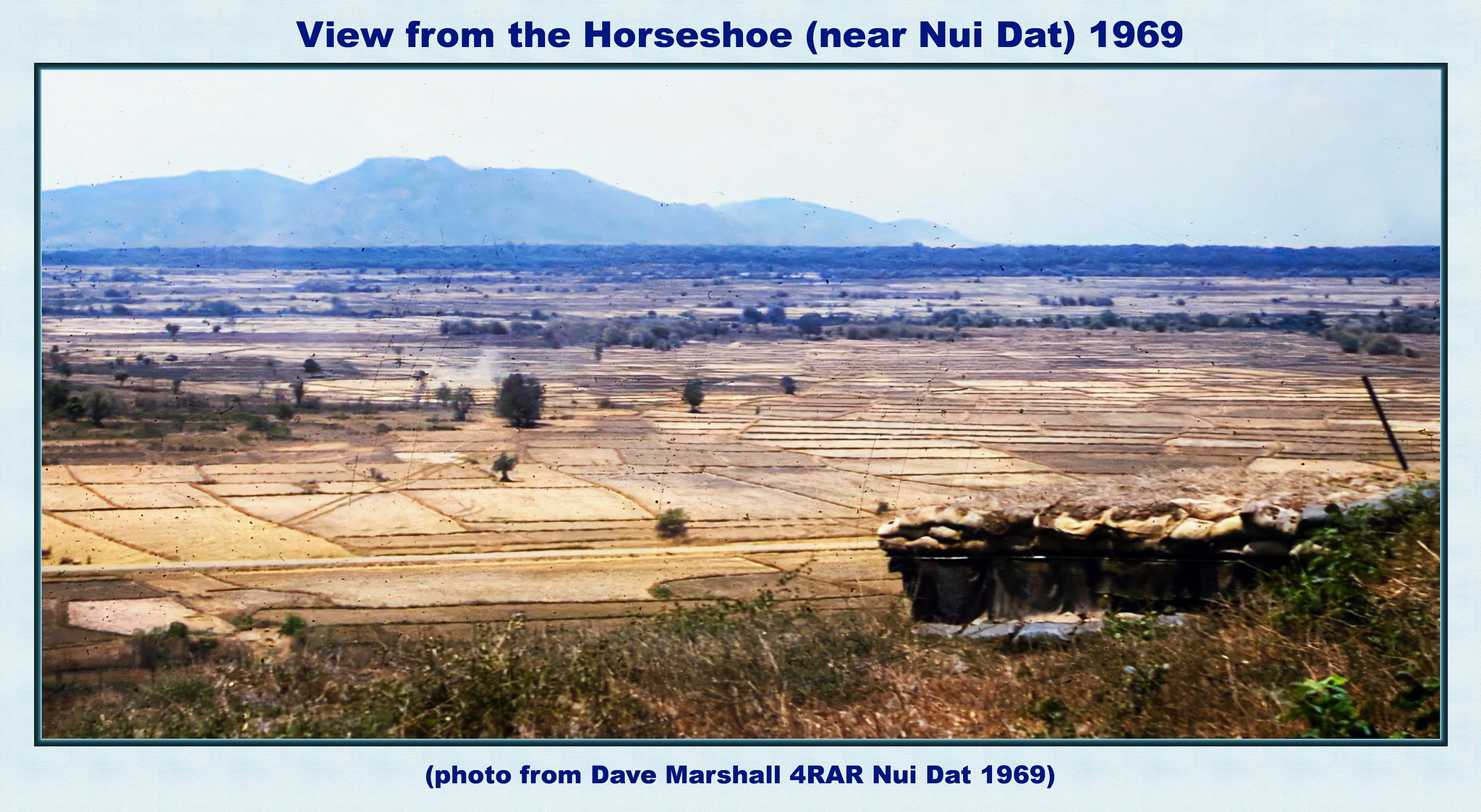This photograph, taken from a hilltop, showcases a vast open plain most likely taken during wartime in 1969 near Nui Dat. The captured ground area is primarily covered in brown soil, segmented by various lines, and sporadically dotted with trees. The scene extends into the background where mountains can be seen, albeit somewhat blurred. The sky displays a gradient from white to light blue on the right side. The bottom portion of the image reveals part of the hill from which the photo is taken, featuring green and brown grass. A small man-made structure, resembling a military post or sandbag bunker, is visible on the right side of the hill. The photo is bordered in light blue with text inscribed in dark blue at the top and bottom. The top reads, “View from the Horseshoe, near Nui Dat, 1969,” and the bottom, within brackets, states, “Photo from Dave Marshall, 4 RAR, Nui Dat, 1969.” The hazy atmosphere and absence of people further evoke the desolation of a combat zone.